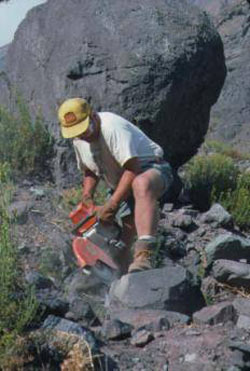In this daytime outdoor photograph, a sunburned Caucasian man stands at the center, slightly bent over with eyes possibly shielded by a yellow baseball cap. He is dressed in a light-colored, short-sleeved shirt, blue jean shorts, and brown work boots with white socks. The man wears brown leather gloves and wields a silver electric saw adorned with red sections on the handle and blade cover. He is actively cutting into a section of gray rock while standing on it. Around him, there is a scattering of green shrubs and brush, particularly dense on the left side of the image. Behind him looms a massive boulder, alongside a collection of other large rocks and additional foliage. The image shows signs of blurriness and JPEG artifacting but clearly captures the scene of a rocky, sunlit landscape with evidence of ongoing excavation or rock-cutting work.